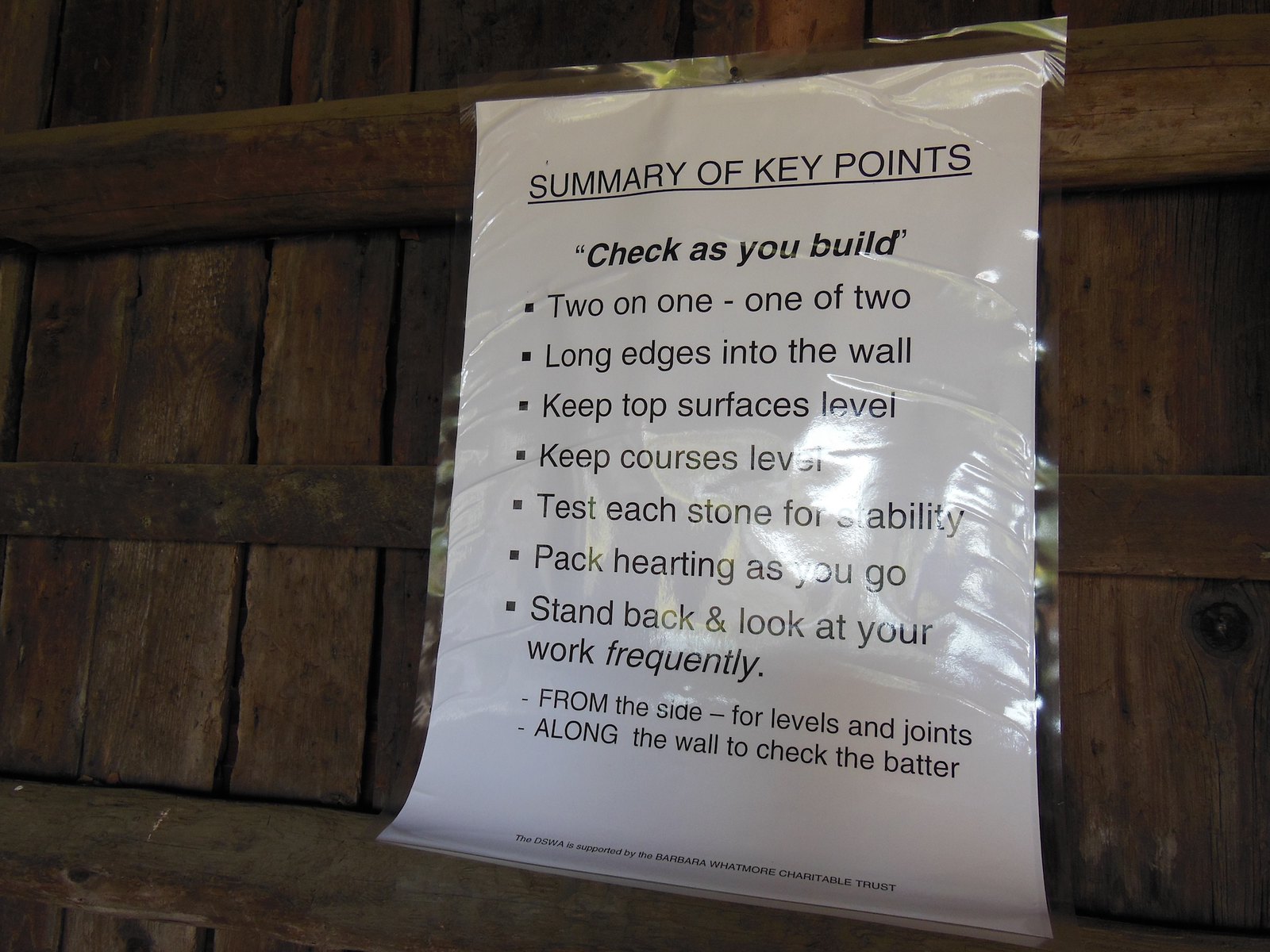A white sheet of paper encased in a clear laminate sleeve is prominently displayed on a wooden wall made of both vertical and horizontal wood panels. The sign, which appears to be secured to the wood either by tape or another adhesive method, contains a neatly centered, black-and-white printed list titled "Summary of Key Points" with the title underlined. The list is structured with bulleted points and includes the note "Check as you build" in parenthesis at the top. The key instructions are:

1. Two on one, one of two
2. Long edges into the wall
3. Keep top surfaces level
4. Keep courses level
5. Test each stone for stability
6. Pack harding as you go
7. Stand back and look at your work frequently from the side for levels and joints along the wall to check the batter.

Additional fine print at the bottom states, "The DSWA is supported by the Barbara Whatmore Charitable Trust." Reflective light on the right side of the laminated sheet suggests the image was captured either with a camera flash or under natural daylight conditions. This detailed instructional sign seems designed for builders working on a structure, providing essential guidelines to ensure precision and stability in their construction work.